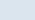A horizontally oriented, rectangular box of silvery blue-gray hue, devoid of any text or imagery. The box’s length is approximately twice the measure of its height. Its calming, understated color is reminiscent of soothing, modern interior decor, making it an ideal candidate for a website background. The soft, serene tone is notably similar to the shade of a bedroom wall, evoking a sense of tranquility and minimalist elegance.